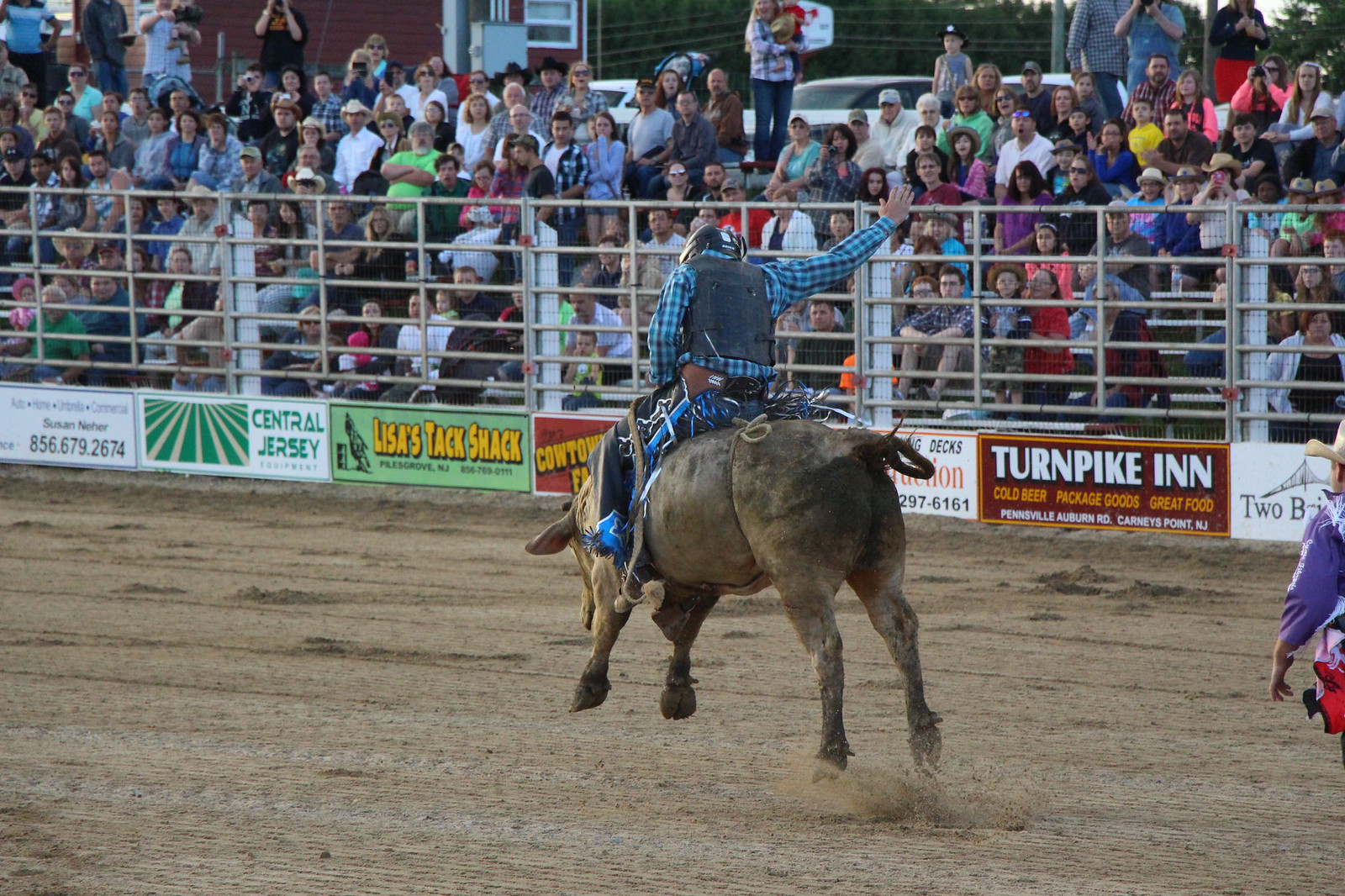In this detailed and vivid image, a rodeo unfolds, capturing the thrilling moment of a bull rider in action. The scene is set in an open-air stadium, surrounded by a backdrop of trees and sky. The focal point is the rider atop a bucking brown bull, both captured in mid-motion with all four of the bull's feet off the ground. The rider, facing away from the viewer, wears a blue plaid shirt, a dark blue vest, a leather belt, and a cowboy hat. His right arm is raised, emphasizing the dynamic movement. A partially-visible metal grate fence encircles the arena, adorned with colorful advertising banners, such as "Central Jersey," "Lisa's Tax Check," "Piles or Files Grove, New Jersey," and "Turnpike Inn, Pennsville, Auburn Road, Carney's Point, New Jersey." Beyond the fence, a large crowd seated in bleachers adds to the vibrant atmosphere, and parked cars are visible further behind them. The arena's surface is a mix of sand and dirt, enhancing the authentic rodeo experience in this moment of photographic realism.